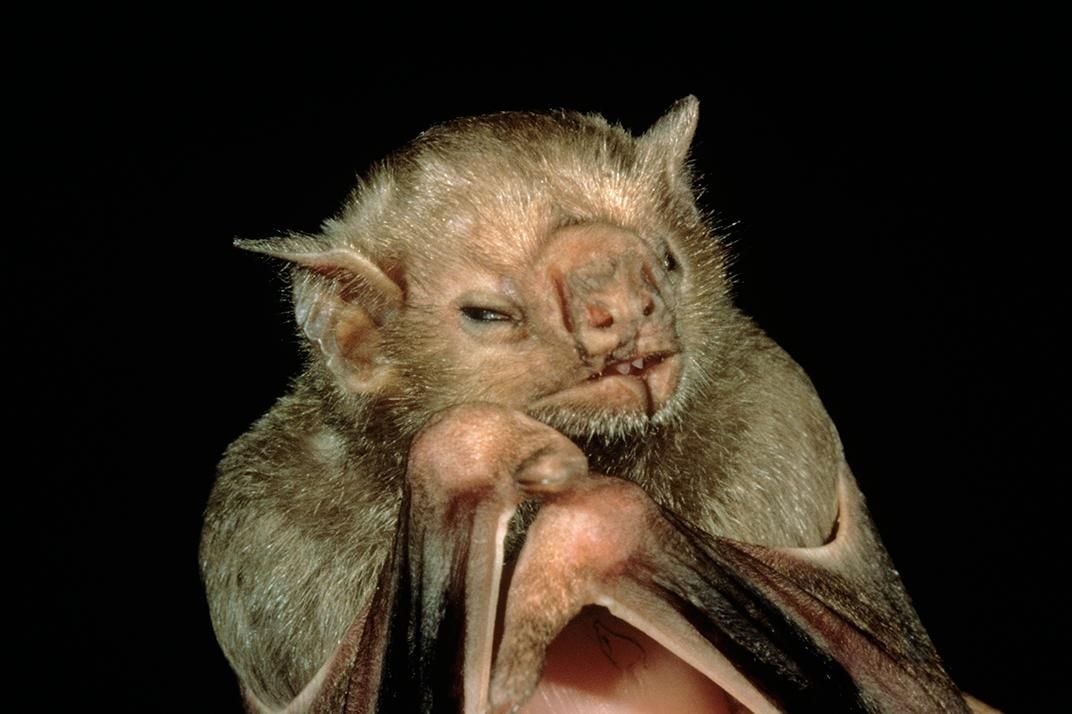In this detailed close-up photo of a bat, set against a stark black background, the creature's face and upper torso are prominently featured. The bat appears as if it has just been roused from slumber, with its slitted, barely open eyes giving it a sleepy or stoned expression. Its fur is light, almost blonde, and slicked back on the head, with shorter hair on its shoulders. The bat's wings are folded up in front of its face, resembling hands, as if it had been napping on its elbows. Its pointed ears extend outward and are pinkish on the inside. The bat's nose is flattened, revealing two nostrils, and its mouth is slightly parted, showcasing two sharp teeth visible from the top. A noticeable scar runs along one side of its face, and a split in the middle of its bottom lip adds to its somewhat rugged appearance. Despite its slightly unsettling features, there is a certain endearing quality to its visage.